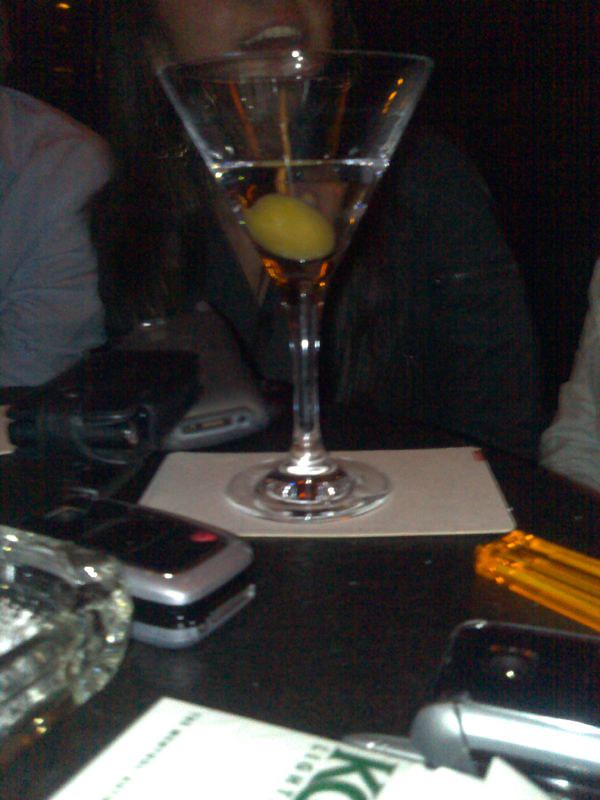This color photograph, likely a low-quality cell phone snapshot, captures an olive martini on a cocktail napkin and a black table in a dimly lit restaurant. The martini, with its toothpick-skewered olive, is the focal point, partially consumed. The table is cluttered with several old-style cell phones, including flip phones and what appears to be a BlackBerry in a leather case. An orange translucent lighter and a cut-off glass ashtray are also present. A partly visible white cigarette pack with the dark green Kool logo is near the martini. Behind the martini glass, the face of a woman in a gray sweater is seen, her mouth open in laughter or conversation, adding a lively human element to the scene. The woman is accompanied by another individual in a light gray jacket, holding a silver, closed cell phone. Despite the graininess and blur of the photograph, the festive atmosphere of the moment is palpable.